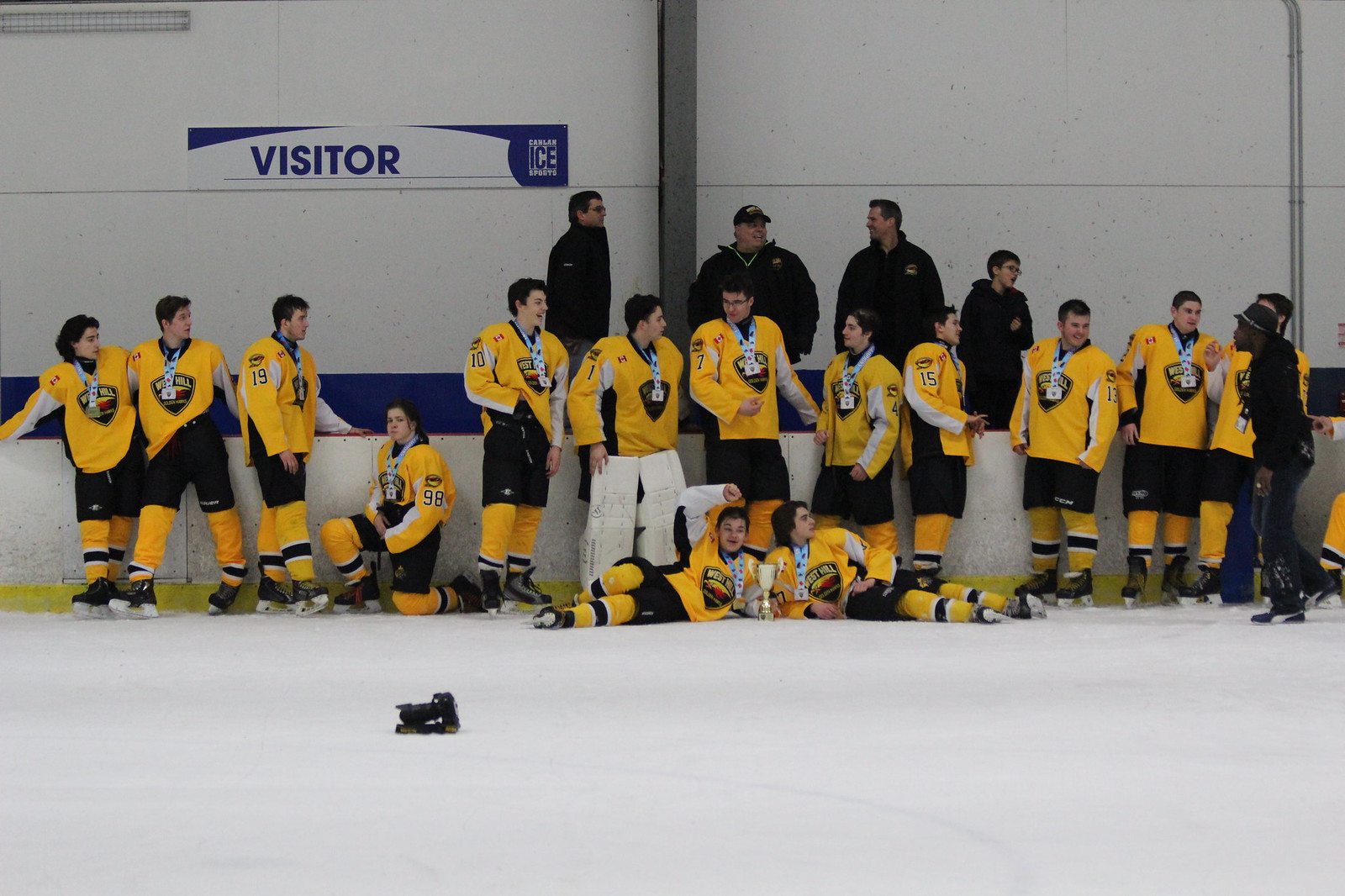In this detailed photograph, a victorious hockey team is assembled on an ice rink for a candid group shot. The players, sporting yellow jerseys with black and yellow pants and skating shoes, are predominantly standing while leaning against a white sideboard marked with a blue sign that reads "VISITOR" and "ICE." Adding to the scene, one player kneels, and two players lie on the ice, shoulder to shoulder, clutching a trophy between them. Their celebratory mood is underscored by the medals around their necks. Surrounding the team are four coaches in black jackets, one of whom sports a baseball cap. The bright, white ice contrasts sharply with the black object, possibly a camera, lying near the center. Above, a tube light illuminates the scene, casting a warm glow on the triumphant players who appear to be in a relaxed, pre- or post-official photo shoot moment, their attention scattered and unfocused on the camera.